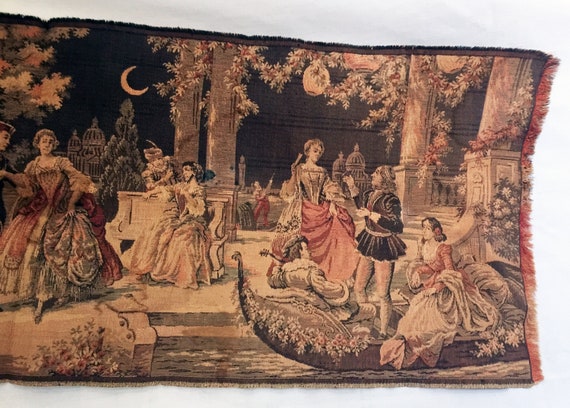The image is of an intricately woven, possibly antique tapestry that vividly depicts a romantic, historical scene set in Venice. Dominating the foreground is a partly flower-adorned gondola floating on a canal. A man standing in the gondola appears to be assisting a woman in an elaborate ballgown with a voluminous skirt, while another man, seated and playing an instrument, is accompanied by a lady who seems to be listening intently. In a scene to the left, a lady on the bench is engaged in conversation with a figure standing behind her. Another woman, almost hidden by the dress she is picking up slightly, stands further left. The background features several grand buildings decorated with lanterns and ivy-draped marble columns, under which the figures stand. Scattered throughout are flowering bushes and plants. Illuminating this serene night scene is a crescent moon positioned slightly to the left, adding a touch of magic to the tapestry's elegant design.